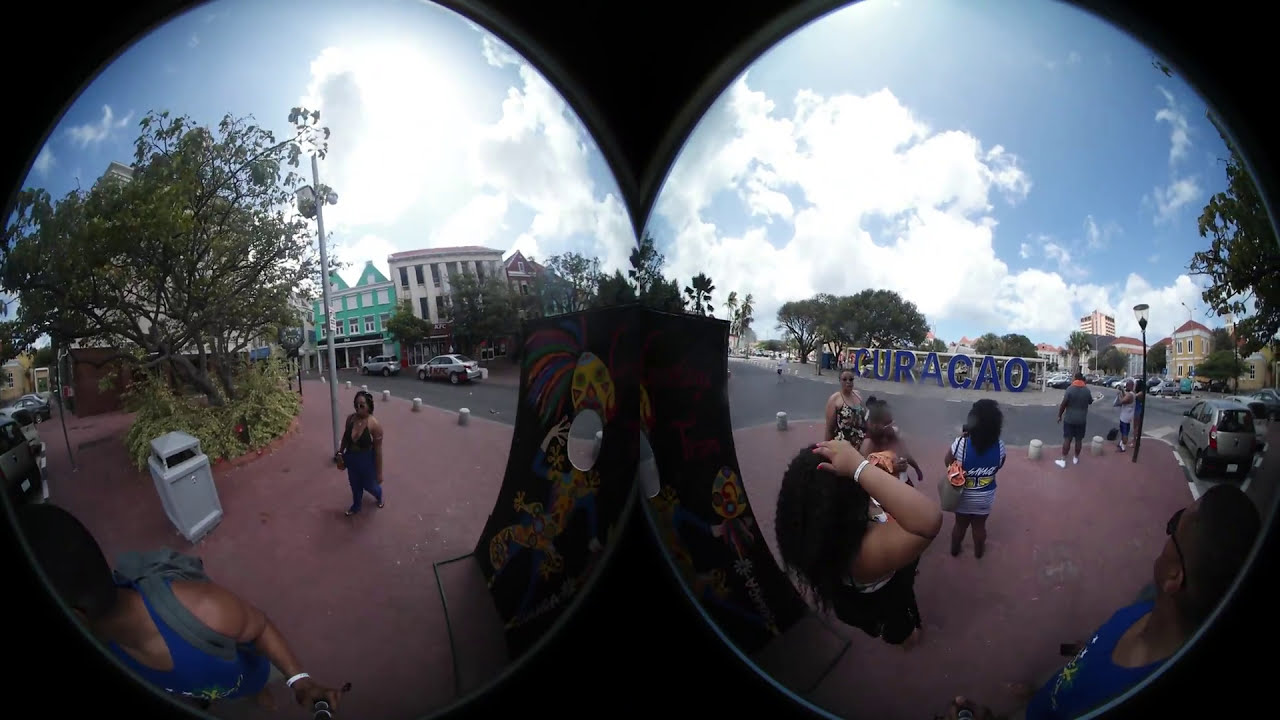The panoramic image, captured through a binocular lens effect, presents a vibrant pedestrian walkway paved with red bricks. The walkway is bordered by short, gray concrete barriers that separate it from a black asphalt road where several cars are parked. The road features a crosswalk and multiple cars waiting to proceed, as well as a prominent blue sign with large letters that spell "C-U-R-A-C-A-O" across the street. A lamppost stands at a corner near the crosswalk, while a rectangular-shaped trash can is visible on the left side.

The left lens of the binocular view captures a scene with a woman in a black bikini top and blue pants holding an object in her hand. A man in a tank top with dark skin appears partially in view towards the front. Behind them, a white trash can is positioned next to a rounded garden featuring green bushes and a large tree. The background reveals two parked cars along with a white and a green building, both with blue and white accents at the top.

The right lens focuses on a group of five to six women gathered on a street corner, standing on the sidewalk and looking out towards the street. The blue "C-U-R-A-C-A-O" sign is clearly visible in this lens as well. The sky above is bright blue, adorned with white, puffy clouds. Various green trees with lush foliage are present in both lenses, adding a touch of nature to the urban landscape. A silver street lamp post is also depicted on the left side of the left oval.

Overall, the image, taken during a sunny day, offers a detailed snapshot of a vibrant urban scene from the perspective of someone peering through binoculars or goggles, seamlessly blending two different angles into one cohesive view.